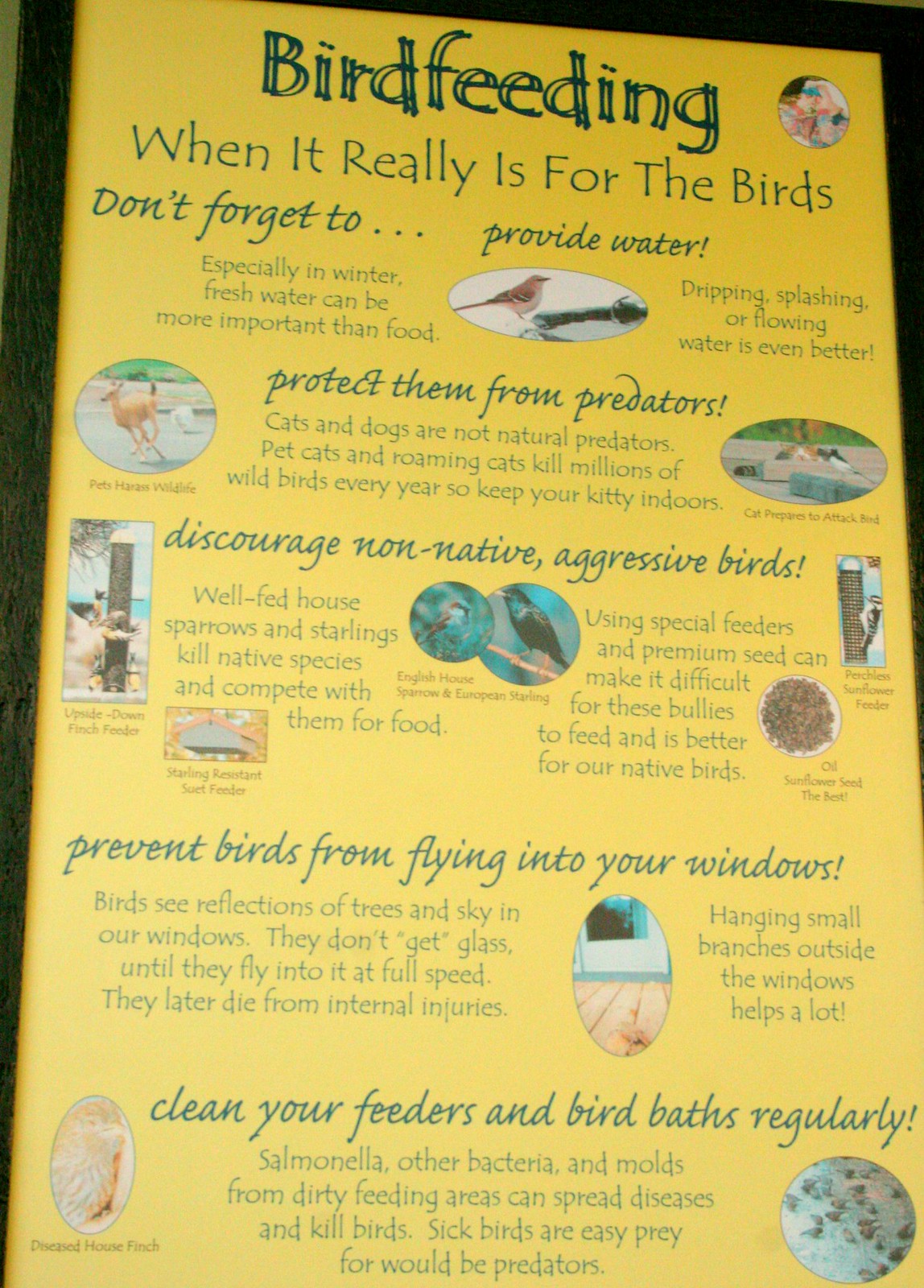This is a photograph of an informational sign that appears to be located in a park or riparian preserve. The vertically long, yellow rectangular sign is mounted on a wooden board, and its text and images are printed directly onto it. At the top of the sign, the title reads "Bird Feeding," followed by the subtitle "When it really is for the birds." The sign details various practices for feeding and protecting birds.

Sections of the sign, written with subtitles in an almost cursive handwriting font, include multiple pieces of advice: "Don't forget to provide water, especially in the winter," emphasizing that fresh water can be more important than food, and noting that "dripping, splashing, or flowing water is even better." Another section advises to "protect them from predators," illustrated with an image of a deer. Additional sections urge readers to "discourage non-native aggressive birds," "prevent birds from flying into your windows," and "clean your feeders and bird baths regularly."

The sign is interspersed with multiple images—mostly ovals, circles, and some rectangles—depicting various birds and related scenes.